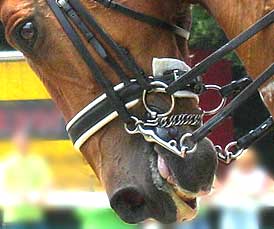This detailed photograph captures a close-up view of a brown horse's head, focusing primarily on the left side of its face. The horse, with big brown eyes and black nostrils, appears to be slightly opening its mouth, with its tongue faintly sticking out. It has a complex bridle arrangement consisting of black leather straps, silver rings, and a chain that extends across the bottom of its jaw. The combination of black straps with embedded silver rings gives the bridle a distinct appearance. Out of focus, the background features blurred images of a few people along with some indistinct yellow and red objects, adding depth to the scene. The horse's calm demeanor is evident in the image, highlighting the intricate details of the tack and the animal's expressive face.